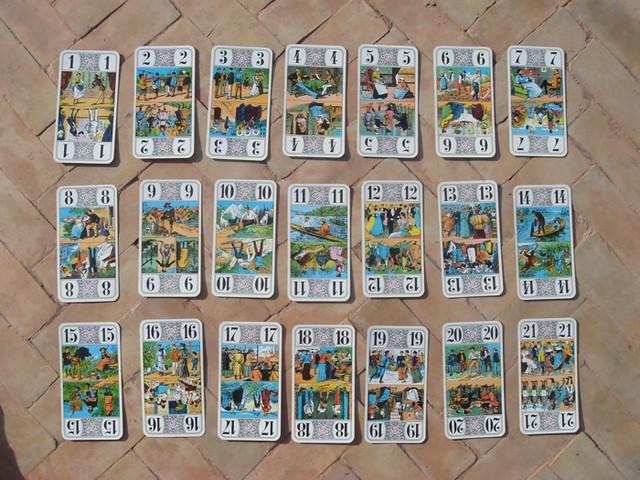The image depicts a detailed, intricate scene set against a light brown, reddish-hued, brick pattern floor. The floor features an alternating pattern with bricks oriented vertically on a diagonal and horizontally on a diagonal, creating a dynamic visual effect. 

On this floor is a series of playing card-sized cards laid out in three rows of seven, making a total of 21 cards. Each card is numbered in all four corners, starting from one and progressing up to 21. The center of each card showcases mirrored illustrations, often depicting a person. One typical illustration features a woman in a dress conversing with another individual garbed in brown and yellow attire, reflecting symmetry and balance. 

The illustrated figures on the cards are adorned in Western-style clothing, showcasing a palette of whites, tans, browns, blacks, as well as occasional blues and yellows. Additionally, some cards depict small, detailed scenes of blue water, green trees, and distant mountains, enhancing the depth and richness of the artwork despite its miniature scale. The overall composition combines both structured patterns and intricately detailed imagery, creating a visually engaging and richly textured tableau.